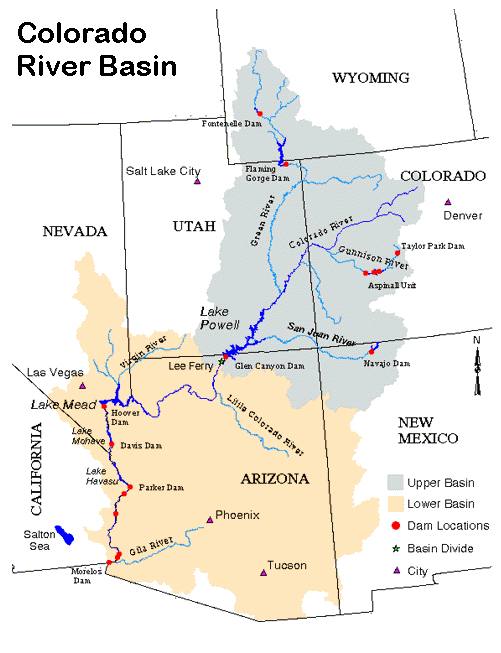The map titled "Colorado River Basin," outlined in black, depicts the detailed geography and hydrology of the region, covering parts of Wyoming, Nevada, Utah, Colorado, California, Arizona, and New Mexico. The rivers are marked in blue, with the Colorado River running diagonally from Colorado through Utah to Lake Powell, near the Arizona border. The map highlights various water bodies, including Lake Mead, Lake Mojave, and Lake Havasu, all situated along the Colorado River.

The upper basin is shaded gray, encompassing river systems in Wyoming, Colorado, and Utah, while the lower basin, colored light yellow, covers areas mainly in Nevada, California, and Arizona. Notable rivers such as the Green River, which intersects with the Colorado River, and the San Juan River, are prominently displayed.

Red dots on the map indicate dam locations, including Flaming Gorge Dam in Wyoming, Taylor Park Dam, Gunnison River in Colorado, and Parker Dam near the Arizona-California border. The map also features black-outlined major cities like Denver, Salt Lake City, Las Vegas, Phoenix, and Tucson, with red triangles marking their locations. Basin divides, symbolized by small stars, are also illustrated, notably at Lee Ferry below Lake Powell.

A key located at the bottom right details the color and symbol codes used: gray for the upper basin, light yellow for the lower basin, red dots for dam locations, stars for basin divides, and triangles for cities.